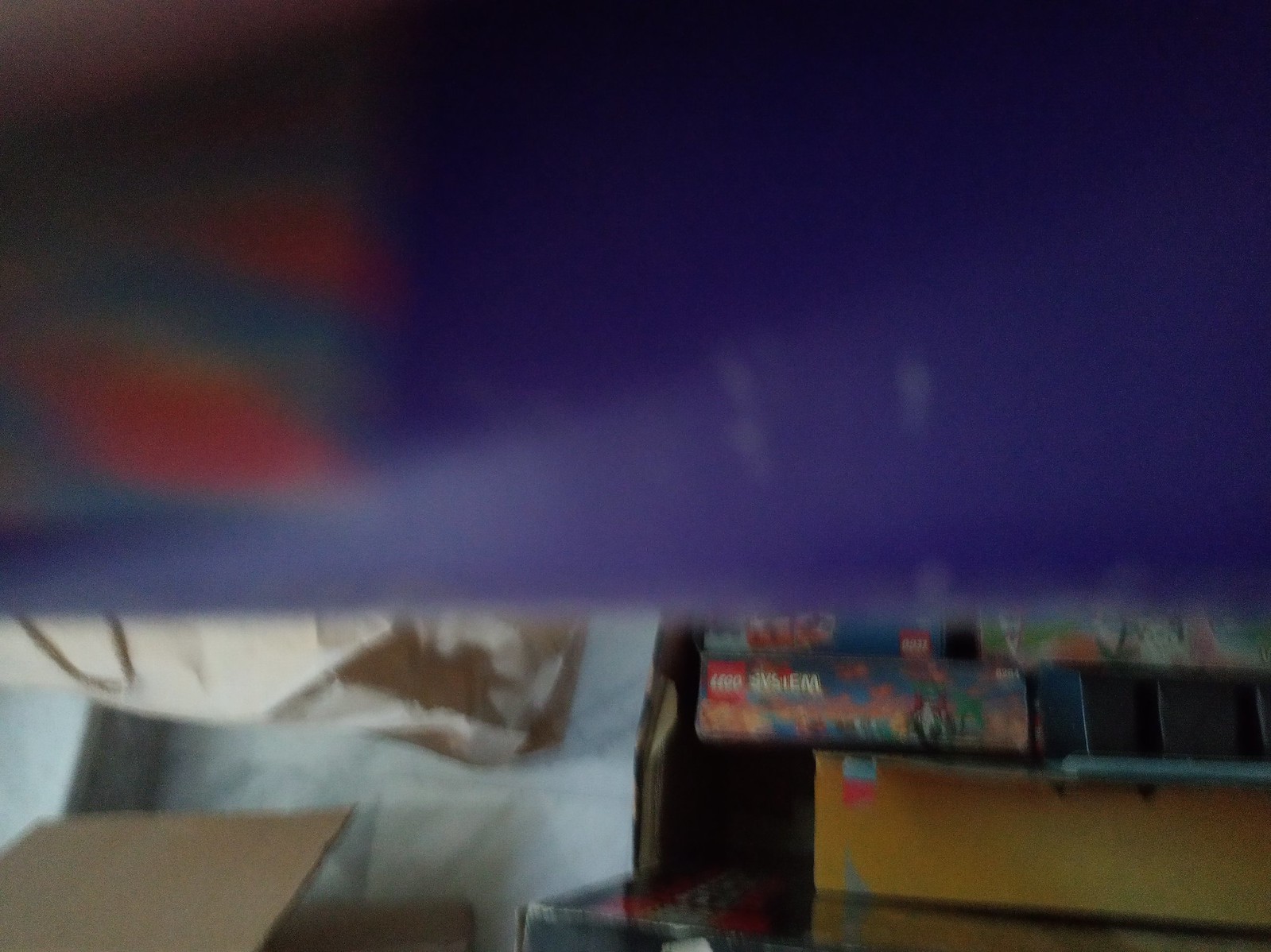The image is significantly obscured, with a large, blurry blue object occupying more than the top half of the frame, suggesting it is very close to the viewfinder and making it indiscernible. In the background, a storage area becomes visible. Various cardboard boxes are scattered, and there appears to be either white flooring or white packaging material. To the right, a stack of Lego boxes is noticeable, with the words "Lego System" visible on one of them. These Lego boxes are placed atop an unbranded cardboard box.